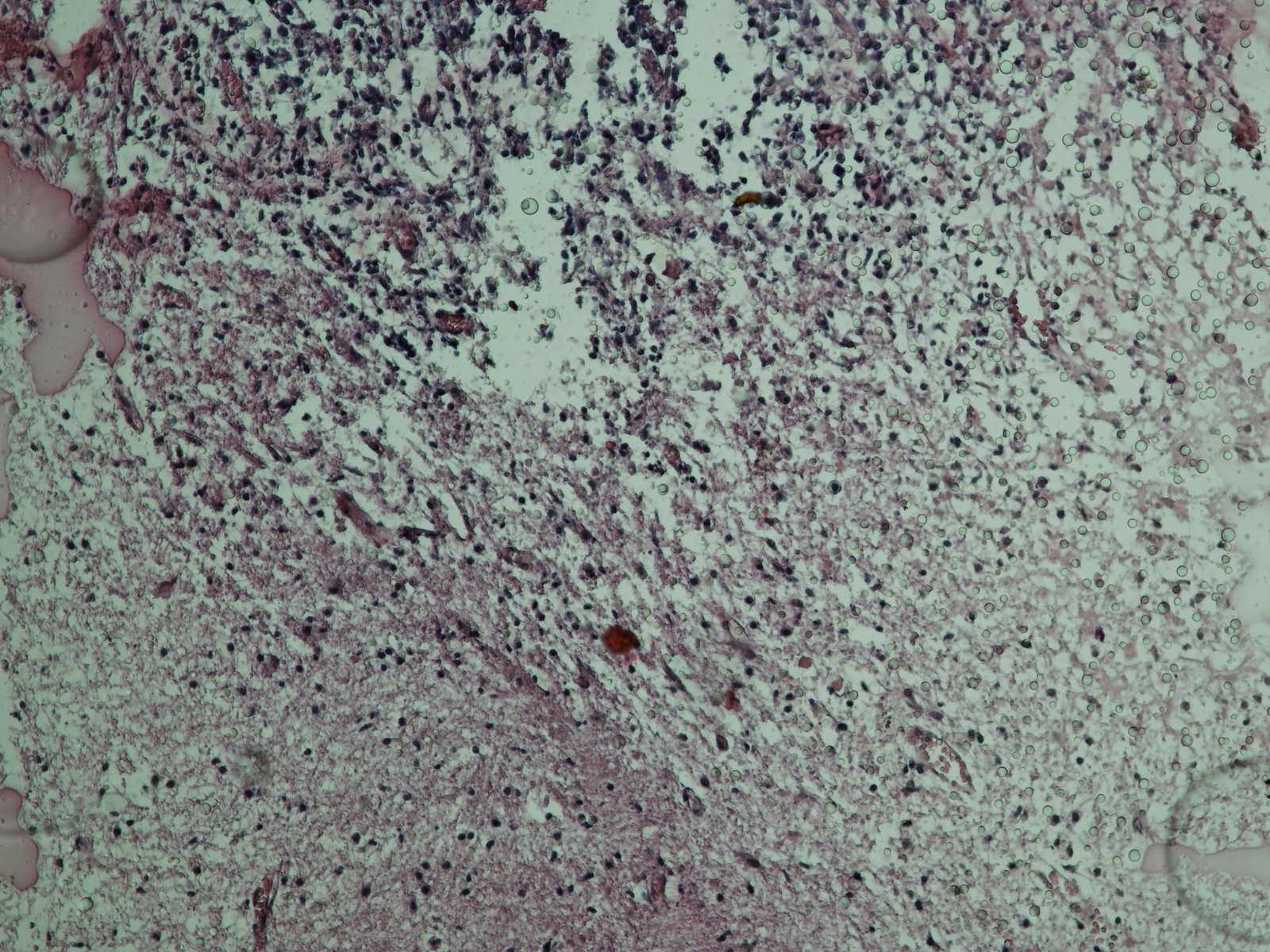The photograph appears to be a highly magnified image of a microscopic slide, likely showcasing a dense colony of bacteria or cellular structures. The background is primarily white, with numerous small, scattered black dots and shapes, particularly concentrated at the top right corner. There are also various red and brown marks dispersed across the image, forming distinct patterns and dots that contribute to an overall unsettling, unappealing appearance. Notably, there are stringy pink elements interwoven throughout the scene, alongside several bubbles, especially visible in the top right area of the slide. Larger, less-defined shapes, including grayish-pink and brown blotches, are noticeable in different regions, with some in the bottom left and others in the center-left towards the bottom. The entire composition is busy and appears unhealthy, likely signifying a vibrant but chaotic bacterial environment.